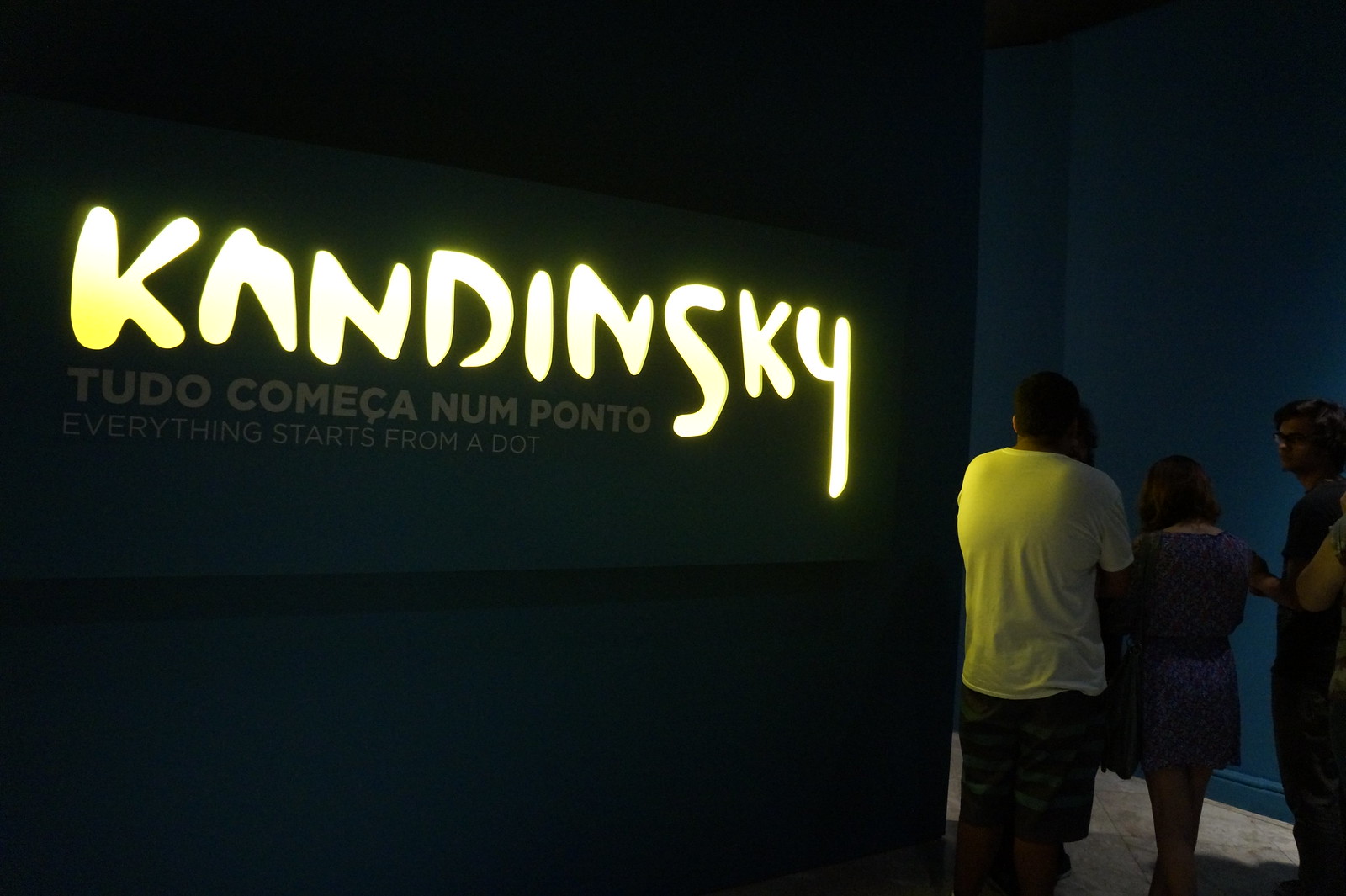The image showcases an indoor scene, likely an art exhibit or museum, during the middle of the day. The floor is composed of stone or tile, and the plain bluish walls frame the setting. In the bottom right corner, three individuals are walking away from the camera towards the exhibit. In the top left corner, a sign reads "Kandinsky, Tudor, Kameka, Nampanto" along with the phrase "Everything starts from a dot." The predominant colors in the image include shades of blue, white, black, gray, and yellow. The focus is on the understated yet informative environment leading to the Kandinsky exhibit, which is highlighted by its lit-up letters.